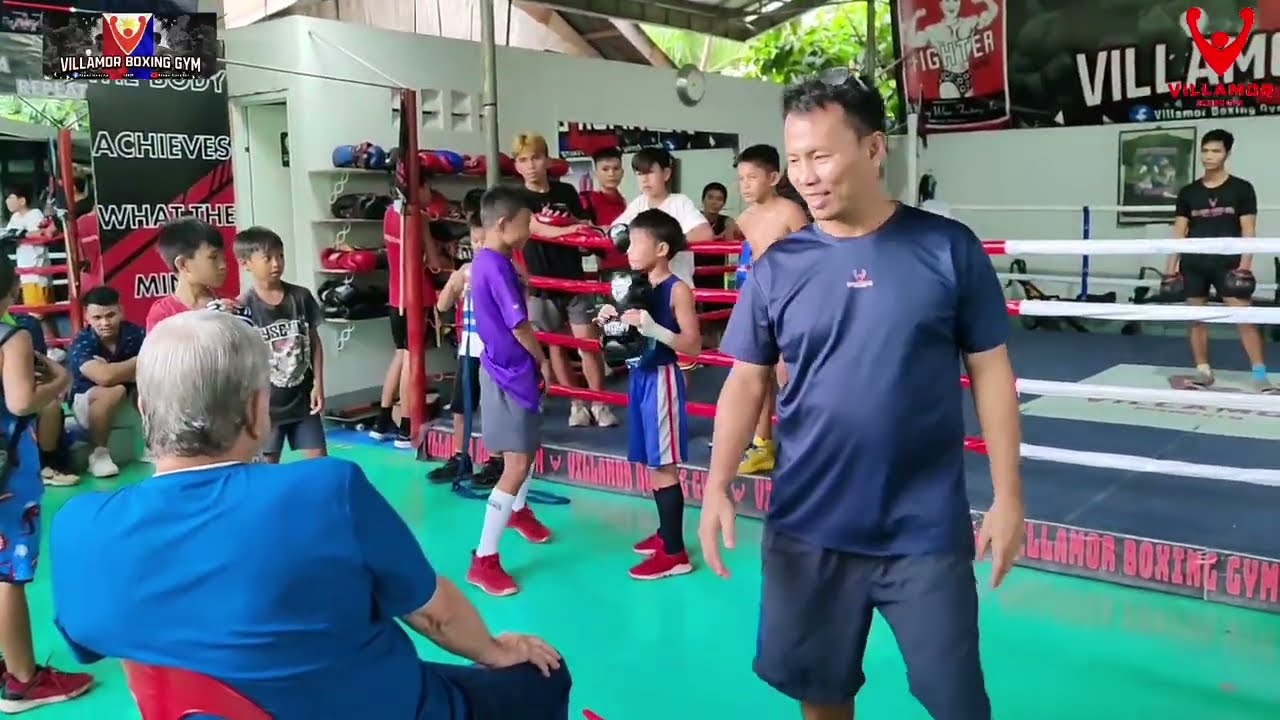The photograph depicts the bustling scene of Villamore Boxing Gym, prominently displayed on a black banner in the upper left corner. The image captures a mix of youth and experience, highlighting a community deeply engaged in training and mentorship. Centered in the image is a middle-aged Asian man with short black hair and glasses resting on his head, dressed in a blue t-shirt and blue shorts. He appears to be in conversation with an older man, who sits on a red chair at the bottom left, identifiable by his gray hair and blue t-shirt. Surrounding them is an energetic group of boys in athletic wear, leaning towards younger ages, likely between 10 and 14 years old, clad in shorts and t-shirts, indicative of a vigorous training session. Behind this assemblage stands a boxing ring, where several older boys seem to be discussing amongst themselves. To the left, a motivational banner partially reads "The body achieves what the mind...", echoing the gym's ethos. The scene vividly portrays the dynamics of training, guidance, and community within this Asian-majority boxing club.